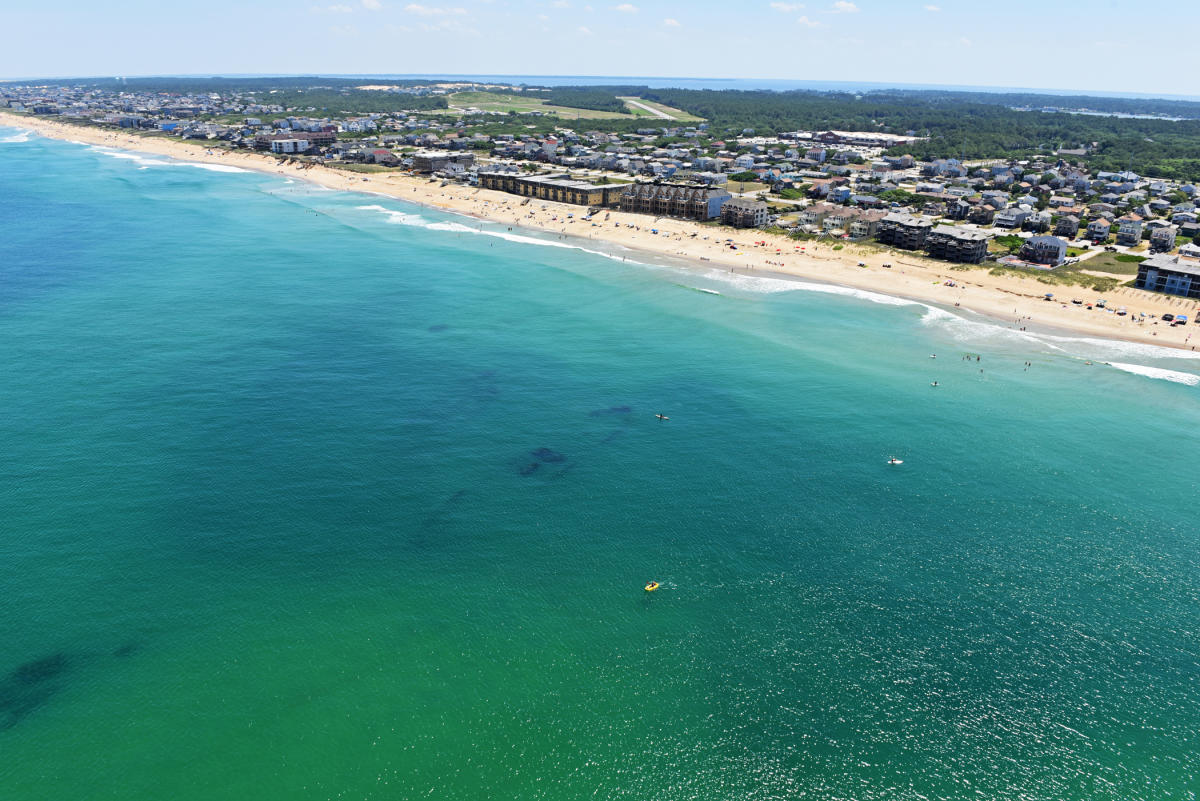This aerial photograph captures a stunning coastal scene with intricate details. Dominating the lower half of the image, the water transitions from a deep green to a bluish-green hue, accented by smooth patches and occasional white tips of waves. The shoreline gently curves from the bottom right, diagonally stretching towards the upper left, where a strip of beige-colored sandy beach is lined with numerous people and umbrellas. Just offshore, several small boats are visible, and one figure on a yellow raft or jet ski stands out.

In the upper part of the image, the scene transitions from the beach to a densely built area featuring an array of low-lying buildings, including condos and beach houses, which extend along the shore and back towards the horizon. This area is interspersed with dark green trees that provide a lush backdrop. Above the buildings, the sky fades into a hazy blue with small, puffy white clouds scattered across it. The land in the background is mostly flat, possibly indicating a thin peninsula with more water on the far side. A road or even an airport runway is faintly visible in the distance. Overall, the photograph offers a comprehensive and vibrant view of a bustling shoreline against a backdrop of calm blue skies and natural greenery.